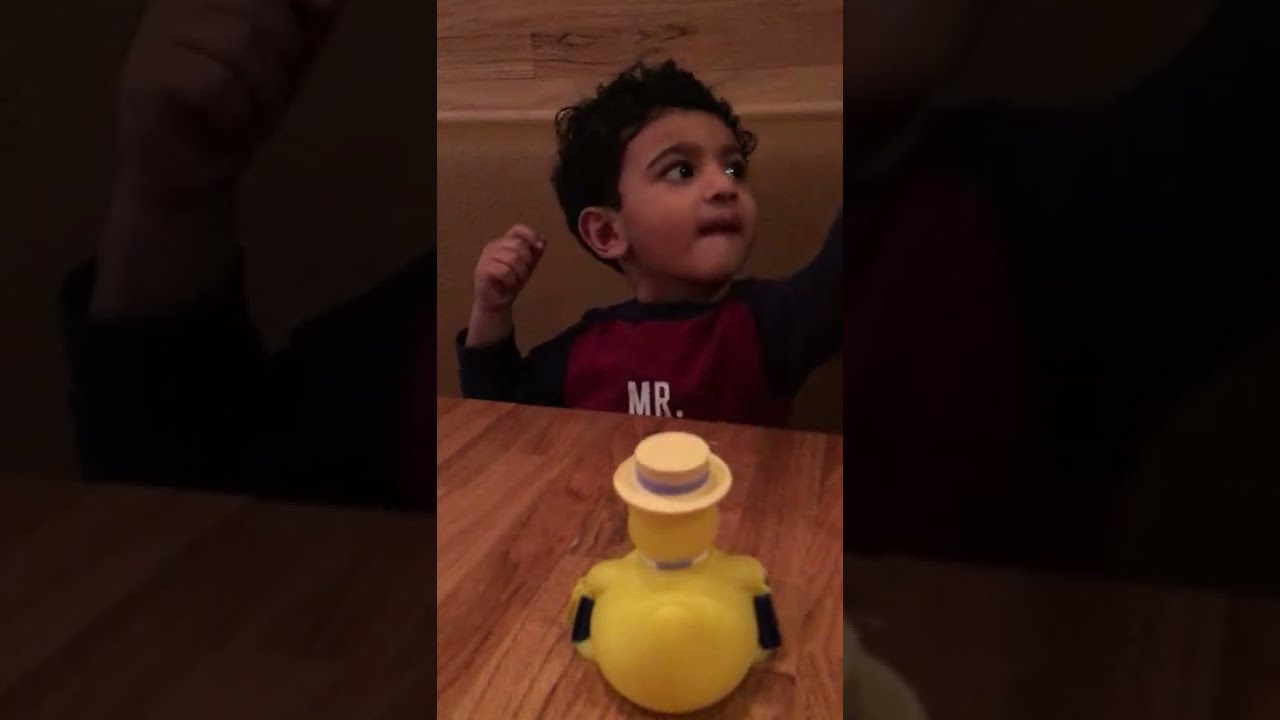The image captures a young child, approximately two years old, seated at a brown hardwood table in an indoor setting. He has short curly black hair and is wearing a red shirt with black sleeves, featuring the text "Mr. M.R." in white prominently displayed in the middle. The child is positioned centrally in the photo, looking off to his left and raising his left arm while his right hand is near his ear. Directly in front of him on the table is a yellow rubber duck, identifiable by its lighter yellow top hat with a purplish ring just above the brim. The background includes an olive-colored booth and walls made of a lighter wood, adding warm tones to the environment, reminiscent of a cozy restaurant setting.